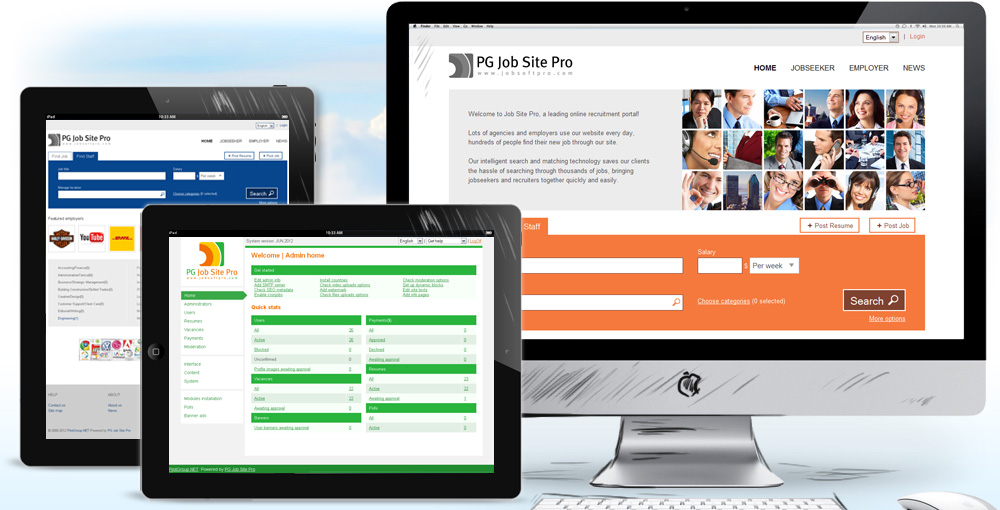In the illustration, we see three devices: a computer monitor and two tablets. On the right side, there is an Apple computer monitor displaying a website with a color scheme of white, dull light gray, and orange. The top-left corner of the website on the monitor features the text "PG Jobsite Pro." 

To the left foreground, a tablet displays a vibrant design with white and green elements on its screen. Behind it, another tablet, oriented in portrait mode, shows a screen with a white background complemented by gray frames and a yellow and red square. All three devices—the computer monitor and the two tablets—feature black frames encasing their screens.